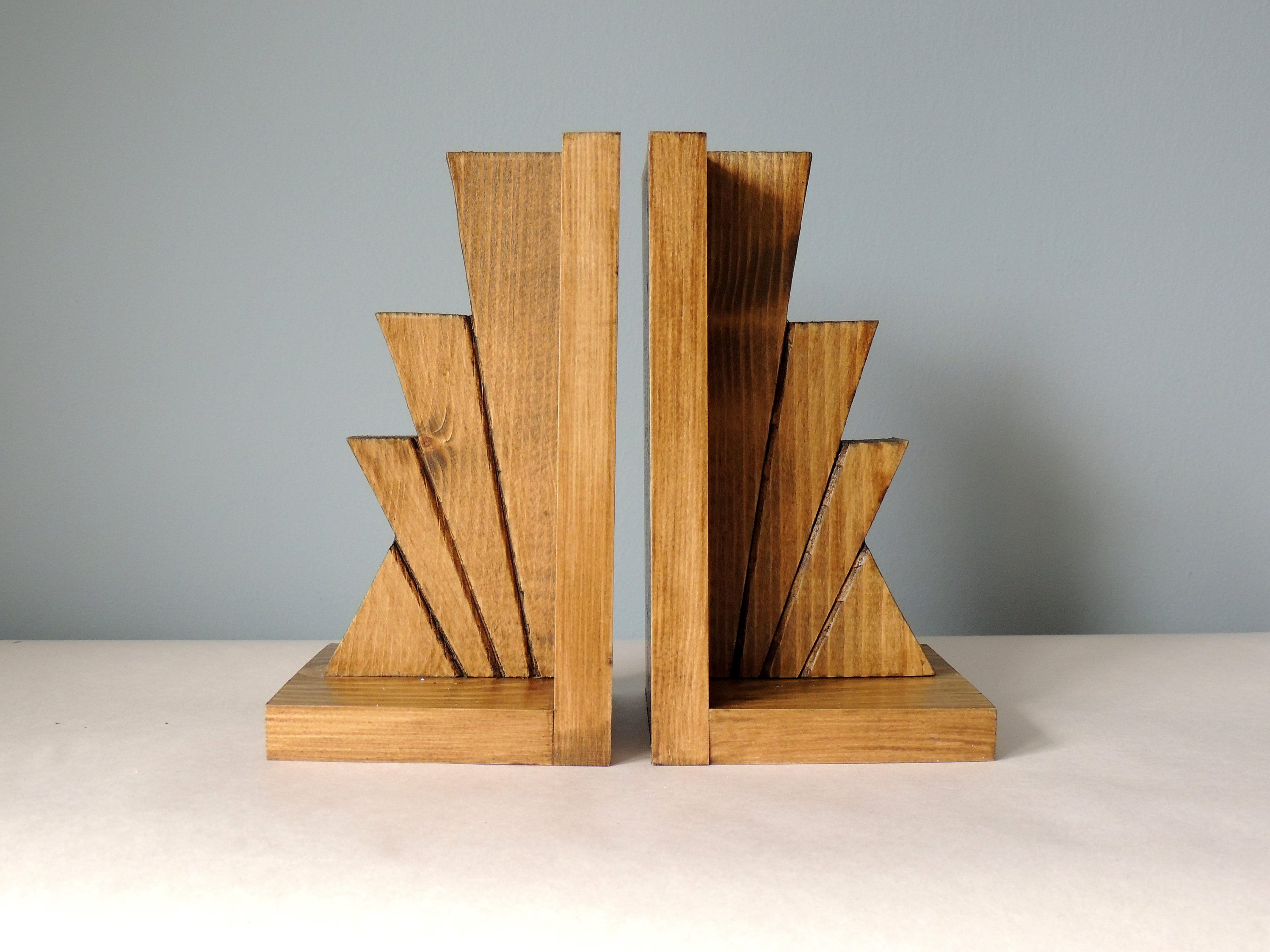The photograph, presented in landscape orientation, captures a pair of wooden bookends on a white tabletop against a grayish-blue wall. The bookends are crafted from medium-toned wood, each constructed in the shape of a backward L and a forward L, creating a symmetrical, mirror-image arrangement. Within the frame formed by these L-shapes, there are four smaller, angular wooden pieces that stand upright. These inner pieces feature a starburst or sunburst pattern with three distinctly darker etched lines, giving the appearance of rays emanating from a central point. The grain of the wood is clearly visible, highlighting the craftsmanship and the stained finish. The lighting is expertly done, allowing detailed visibility of the wood's texture and the subtle shadowing of the right bookend. This minimalist setup emphasizes the intricate design and the natural beauty of the wood grain, suggesting a catalog-style presentation focused solely on the bookends without any additional elements in the frame.